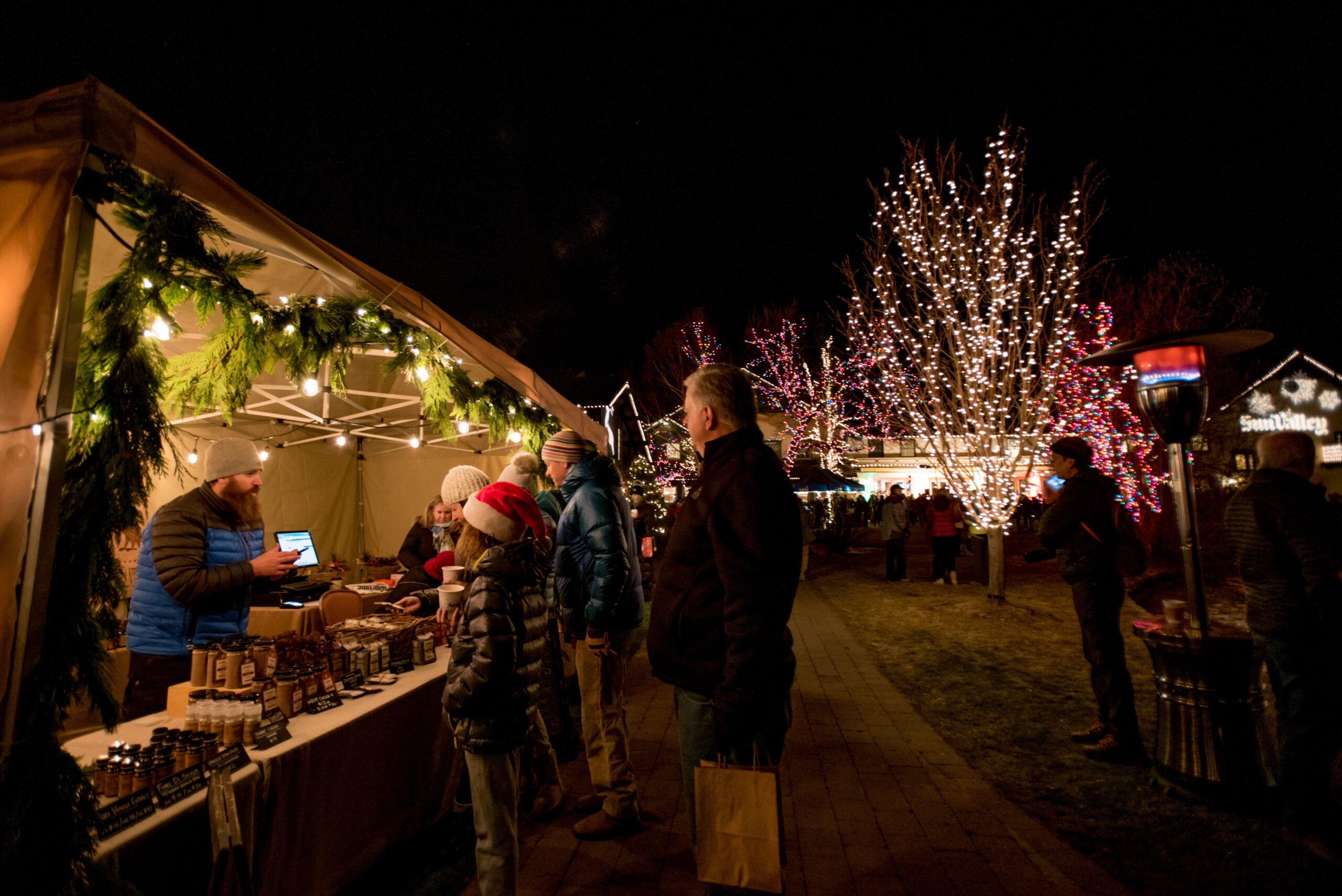The image captures a festive nighttime scene at a bustling Christmas market illuminated by numerous lights. In the foreground, a man dressed in a black and blue puffer jacket, sporting a long beard and a toboggan hat, tends to a tent decorated with pine boughs and green Christmas garlands. He appears to be selling items, possibly chutneys and jams, as he engages with potential customers gathered around his long table laden with products. Not far from him, a little girl donning a Santa Claus hat stands in her winter coat, adding to the festive atmosphere. The pathway in front of the booth is a brick walkway, lined with several other booths. In the background, trees adorned with white and pink Christmas lights twinkle against the dark, black sky. A building reading "Sun Valley" suggests that this market might be set in Sun Valley, Utah. The scene is lively with numerous people wandering, warmly dressed, some holding shopping bags and perusing other sellers' stalls, all contributing to a joyful holiday ambiance.